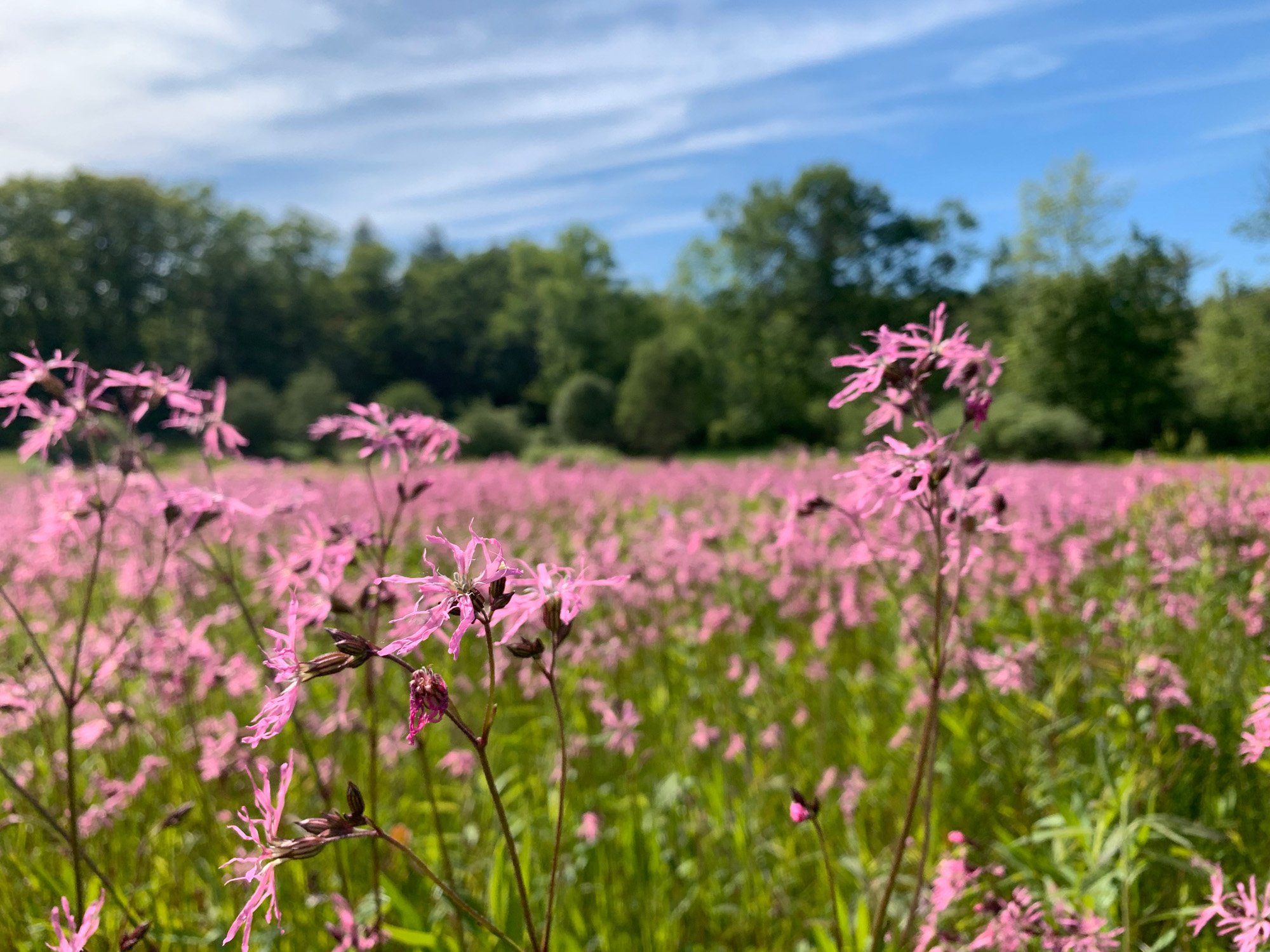A vast field of wildflowers, all of the same rosy pink hue, fills the image. The pink flowers are neither too light nor too dark, striking a balanced, medium shade of pink. The camera's focus is sharply on a few delicate blooms in the foreground, leaving the rest of the image softly blurred to create a dreamy effect. This blurring hints at the expansive field that stretches several feet into the distance, where you can make out the outline of green bushes and trees. The small, delicate blossoms, though numerous, would feel light and dainty if held in your hands, emphasizing the lightness and airy beauty of this pink wildflower meadow.